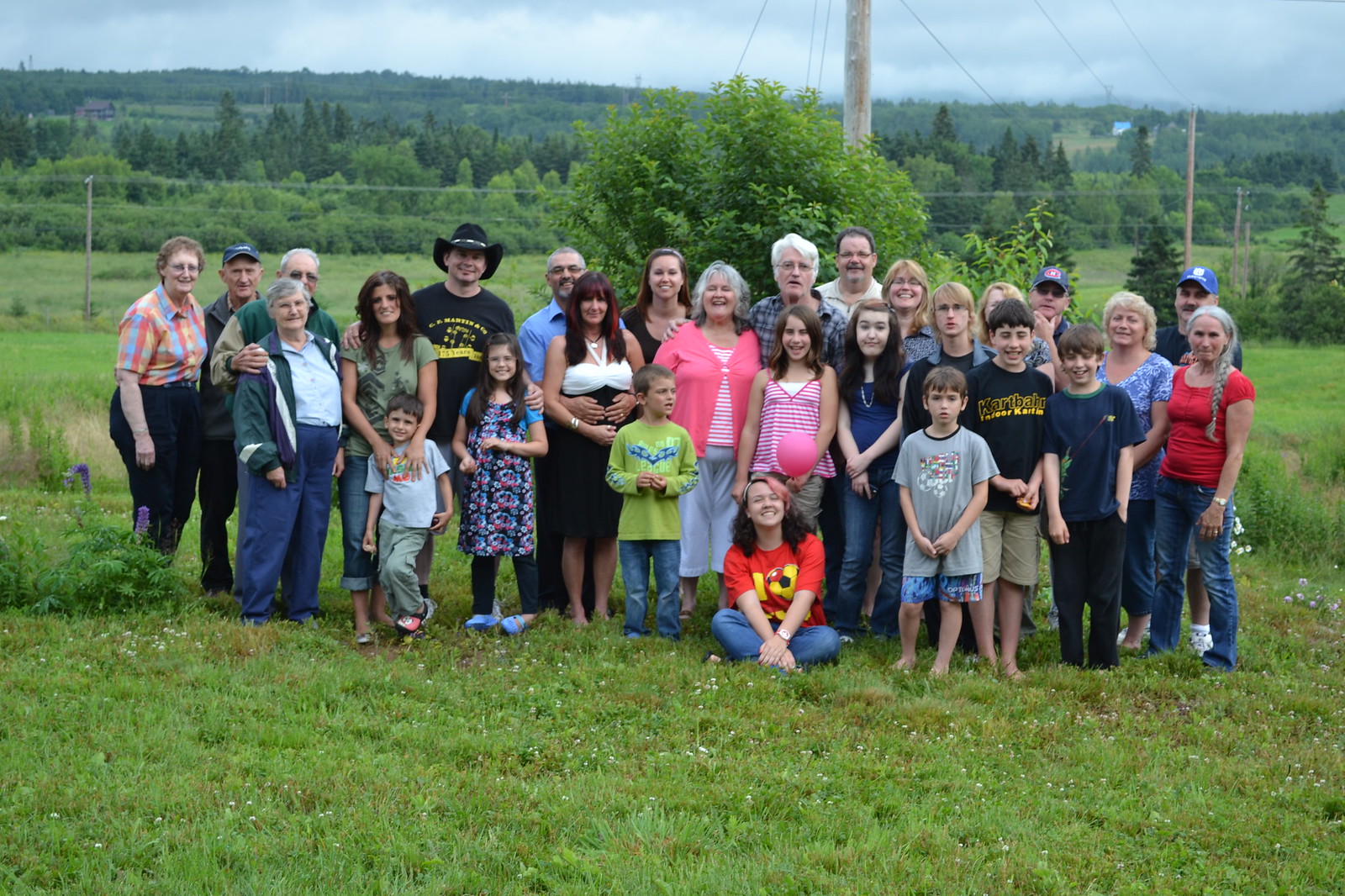This is a detailed group photograph of what appears to be a very large, extended family, spanning several generations. At the center of the image is an elderly couple in their 60s or 70s, surrounded by younger family members, including middle-aged couples, young single adults, and numerous children. The group is arranged in a semi-organized manner, with children standing in the front, some holding items like a ball and a pink balloon. The photo is set in a green, grassy field with sporadic blooming flowers and a backdrop featuring shrubbery, a bushy tree, and distant hills. The sky is cloudy and gray, adding a subdued tone to the scene. Various family members are dressed casually in blue jeans, black pants, shorts, and t-shirts, while a few sport accessories like baseball caps and a cowboy hat. The distant landscape includes utility poles and possibly a tower, suggesting they are in a rural or foothill area. This outdoor daytime photograph captures a moment of togetherness for this diverse, multi-generational family.